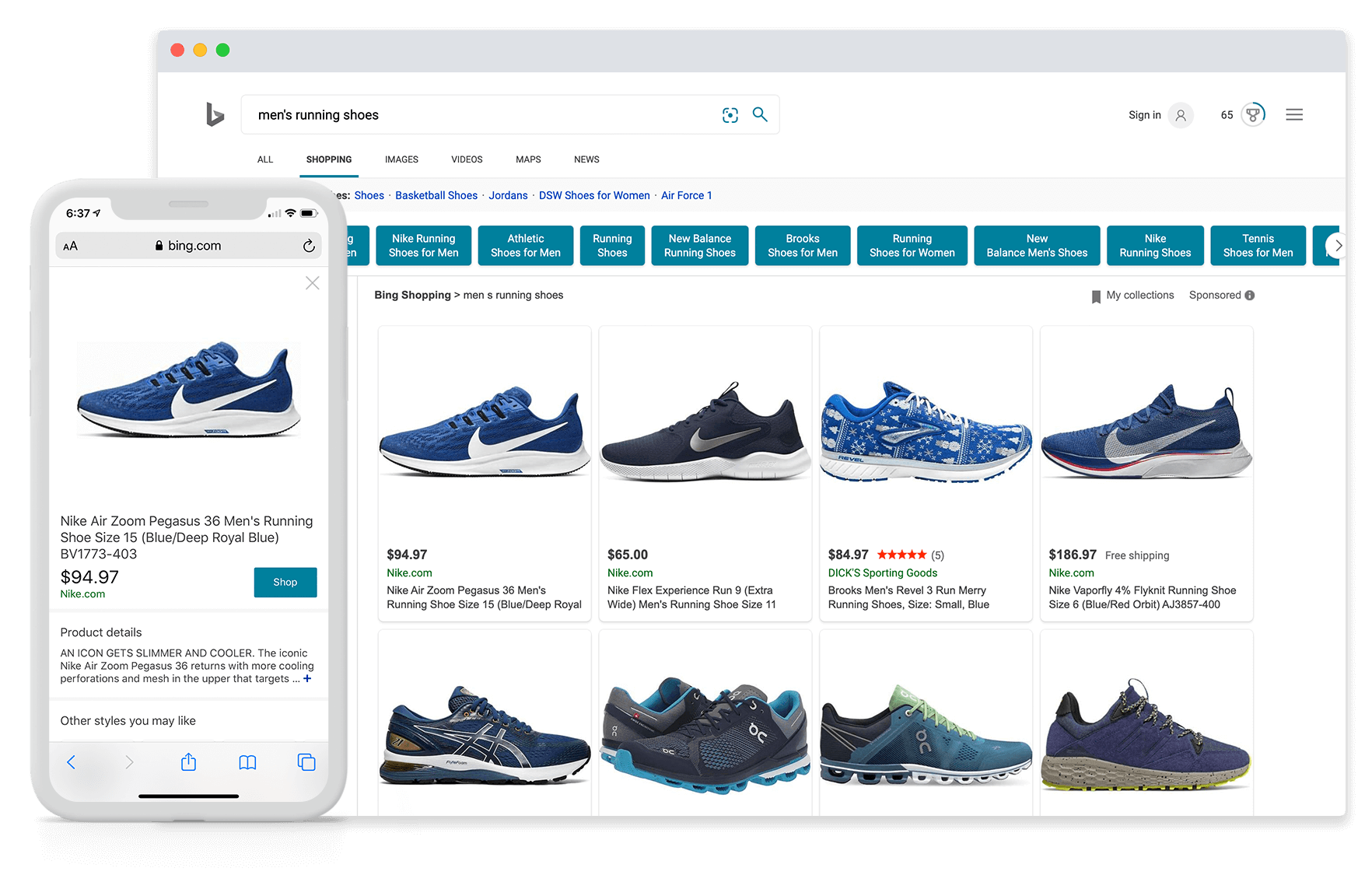This image presents a detailed mock-up comparing Bing search results for "men's running shoes" on two devices: an iPhone and a MacBook. The screenshot captures the distinct window designs characteristic of macOS, with red, yellow, and green dots in the upper left corner. Both platforms display the Bing shopping interface, highlighting a search primarily yielding blue Nike running shoes, despite the color not being specified in the search terms.

On the iPhone screen, a single product—blue Nike sneakers priced at $94.97—is prominently displayed. The MacBook's larger screen features an extended view, showing this same sneaker at the top, followed by additional blue Nike running shoes. A few non-Nike brands are visible towards the bottom, but the top row is entirely dominated by blue Nike footwear.

The Bing logo, positioned towards the top left corner, is understated in black and white, partially obscured by the overlapped devices, suggesting it is not the focal point of the image. This mock-up seems to be crafted to illustrate the visual consistency and presentation of Bing search results across mobile and desktop platforms, though the exact purpose remains unclear.